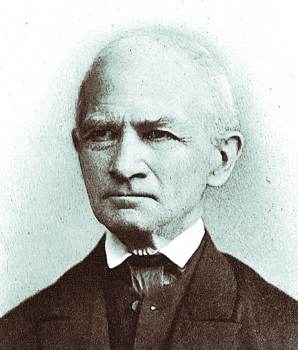This is an old black and white photograph, likely from the early 1900s, depicting an older Caucasian gentleman with a very stern and grimaced expression. His hair is extremely sparse and thin, almost appearing as if he is balding, with what little remains being gray. He has a very short buzzed haircut. His bushy, dark eyebrows are furrowed, emphasizing his stern look. He has a larger nose and thin lips, and his right eye appears to be slightly off-center, facing a little to the left. The gentleman is dressed in a formal, three-piece suit consisting of a black jacket that seems to overwhelm his thin neck, which is further accentuated by a tightly pulled collar and a white collared shirt. The collar is stiff and high, possibly held by a band, and underneath, he wears a vest that buttons up all the way. His ears are average-sized but set low, adding to his distinguished appearance. The photo has a white and gray background, enhancing the contrast and detailing in his features and attire.